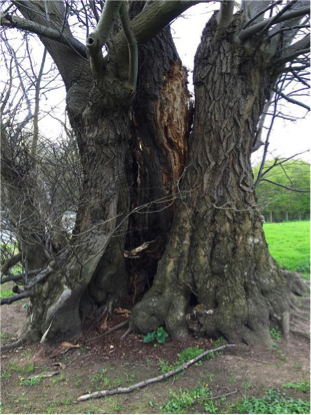The photograph depicts a large, intriguing tree situated outdoors. The tree is especially notable for its unusual appearance, as it seems to have been split in half, possibly by lightning or another force. On closer inspection, it's unclear if it's actually two trees growing closely together or a single tree that has split down the middle. The left side of the tree is significantly larger and appears more robust, while the right side is smaller and looks more lifeless. There is an abundance of roots protruding from the ground at its base, along with branches scattered around and a mix of dirt and sparse grass. No leaves are visible on the tree, emphasizing its barren state. In the background, a patch of green grass is visible along with a distant tree line. The sky above is light blue or gray, giving off an overcast impression, which adds to the somber atmosphere of the scene.